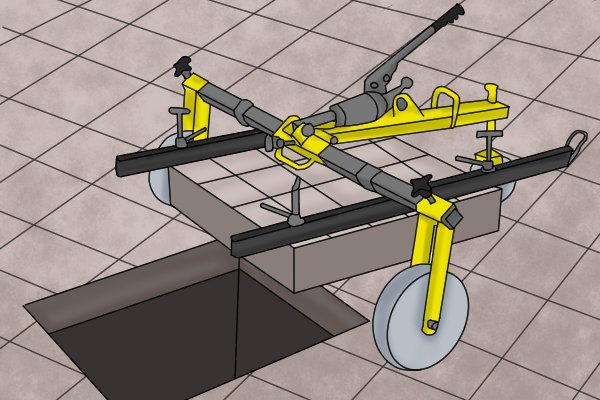This detailed, color illustration presents a digital rendering of a sophisticated machine designed for moving flooring tiles. Positioned on a tiled floor with a pattern of gray grout crosshatching over a tan background, the scene features a large rectangular hole in the lower-left corner of the image. This hole appears deep and is brown at the bottom.

Set slightly off-center toward the right, the machine itself is a complex gray and yellow metal apparatus. It consists of three gray wheels arranged in a triangular pattern and several parallel bars. Additionally, it includes a bar across with a wheel on each side. The focal point of the device is a set of clamps holding a large block, which has the same pattern and color as the floor, suspended above the rectangular hole, creating the impression that the block is about to be inserted into the hole. The machine's design, which includes gray and yellow metal components, emphasizes its industrial function, hinting that it could be utilized in various settings, whether a workplace or a home project. The lack of centering in the composition adds to the dynamic nature of the scene.